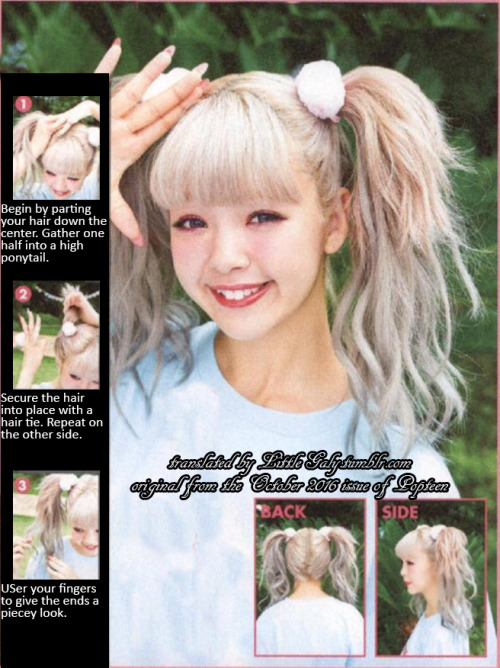In this vertically-oriented image, a teenage or young adult girl with light skin and blonde hair styled into two pigtails and bangs is the central focus. She is outdoors, framed by green grasses, bushes, or trees in the background, and she is smiling directly at the camera while holding up her hand, showcasing long nails. She wears a blue shirt. The image contains layered instructional elements: on the left side, three vertical panels provide a step-by-step guide to replicating her hairstyle, using red numbered circles (1, 2, 3) to indicate the sequence—beginning with parting the hair down the center and creating high ponytails, followed by securing the ponytails with hair ties, and finally, giving the ends a 'piecey' look. Additionally, the bottom right side of the image features two smaller pictures labeled in red font, "back" and "side," showing the back and side view of her hair, respectively. Central text, in black, reads "Translated by littlegayleefumbler.com" with the original source being the October 2016 issue of "Popstein."